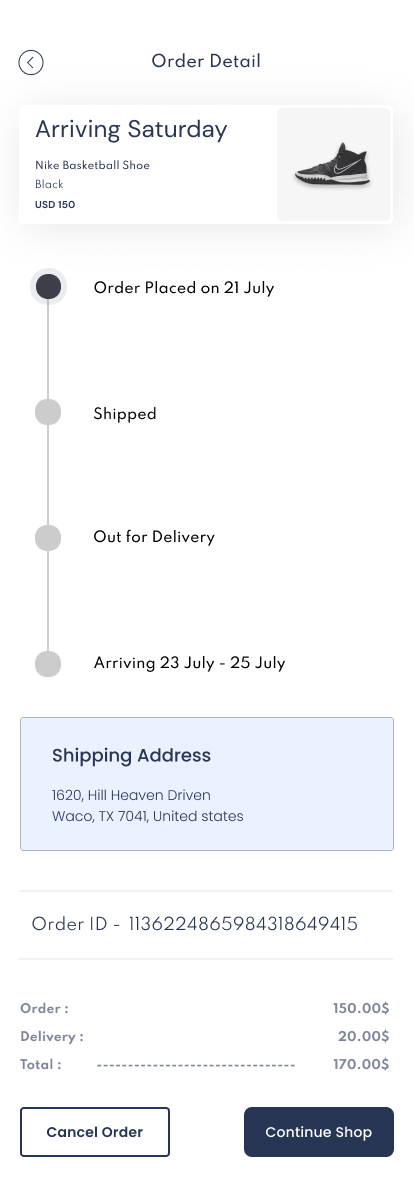The image features a clean, white background with a noticeable order summary prominently displayed. 

At the top center of the image, there is a bold, dark blue text that reads "Order Detailed." 

On the left side of the image, there's a product description reading:
"Arriving Saturday: Nike Basketball Shoe, Black, USD 150."

To the right of this text, there is an image of a black Nike basketball shoe facing left, adorned with a white sole and a white Nike logo.

Beneath the product information, there's a vertical progress bar on the left side with various milestones:
"Order Placed on 21 July" (highlighted in blue) is the first dot.
"Shipped" 
"Out for Delivery"
"Arriving 23 July to 25 July"
The subsequent dots are grey, indicating future steps.

Immediately below the progress bar, there's information set against a light blue background:
"Shipping Address: 1620 Heaven Drive, Waco, TX 741, United States"
"Order ID: 1136224865984318649415"
"Order: $150"
"Delivery: $20"
"Total: $170"

At the bottom of the image, there are two buttons:
A white "Cancel Order" button on the bottom left.
A dark blue "Continue to Shop" button on the bottom right.